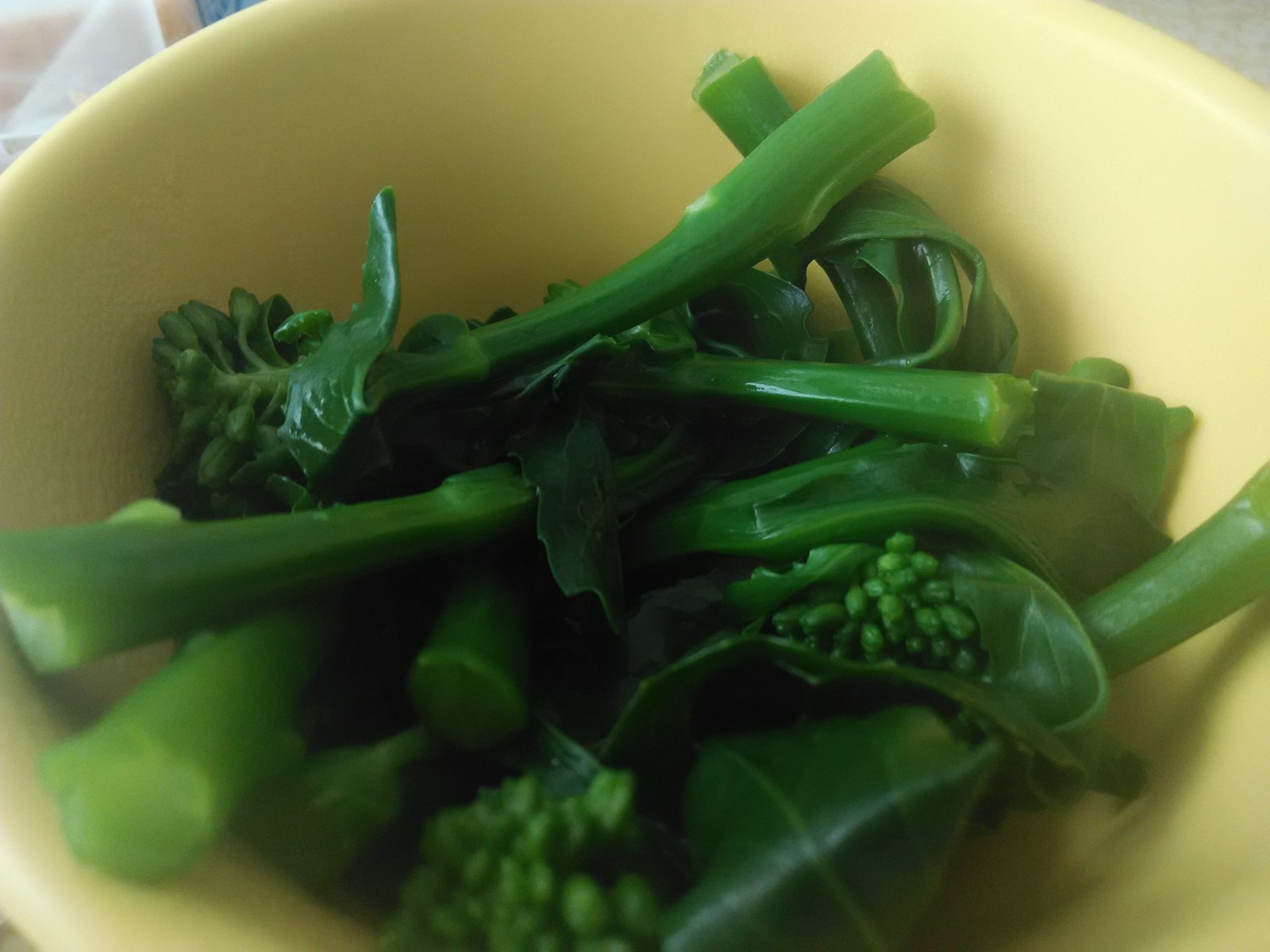This is a close-up color photograph of a bowl filled with bright green broccoli rabe, cooked to a tender, lightly blanched or steamed state. The vegetables, a mix of leafy greens and small seed pods, are casually arranged in a light yellow bowl, their vibrant hue enhanced by the absence of any visible sauce or seasoning. The broccoli rabe casts subtle shadows along the sides of the bowl, contributing to the composition. The bowl itself takes up most of the image, with just the edges of a tablecloth or napkin peeking through the top left and right corners of the frame. The glistening quality of the broccoli rabe suggests it has been recently washed or processed, adding a fresh and appetizing sheen to the dish.